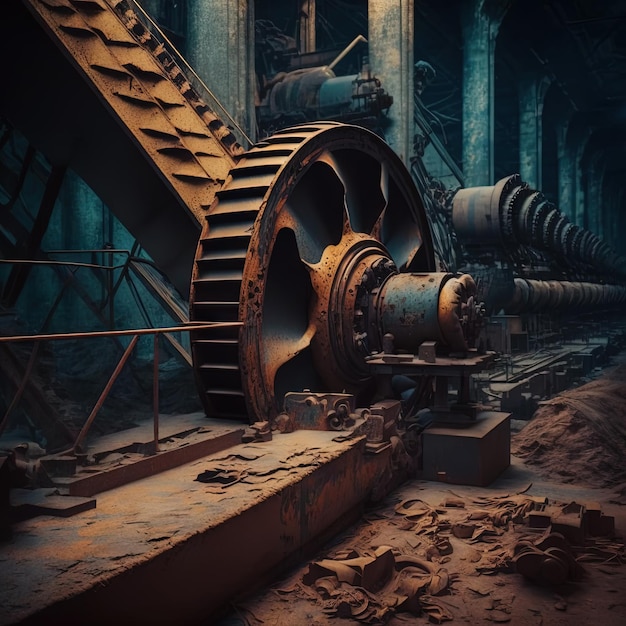The image is an AI-generated, surreal depiction of an abandoned, post-apocalyptic facility, combining elements of a mechanical mill and futuristic turbines. Dominated by shades of rust and turquoise, the scene features a colossal, rusted wheel, reminiscent of a mill wheel, now decrepit and covered in scales of rust. This giant wheel, which once may have powered machinery, sits on a turquoise-blue platform. Surrounding this central wheel are more turbines, arranged diagonally in a line, varying in size and progressively smaller as they recede into the background under dim, minimal lighting. The setting appears to be an immense, deserted warehouse or factory, with towering pillars of metal, steel, or concrete stretching from floor to ceiling. Debris and machinery parts are scattered all over the dirt-colored floor, enhancing the abandoned and decayed atmosphere. The entire environment, shrouded in darkness, suggests the scene could be either underground or cloaked in the night, adding to its haunting, dystopian essence.